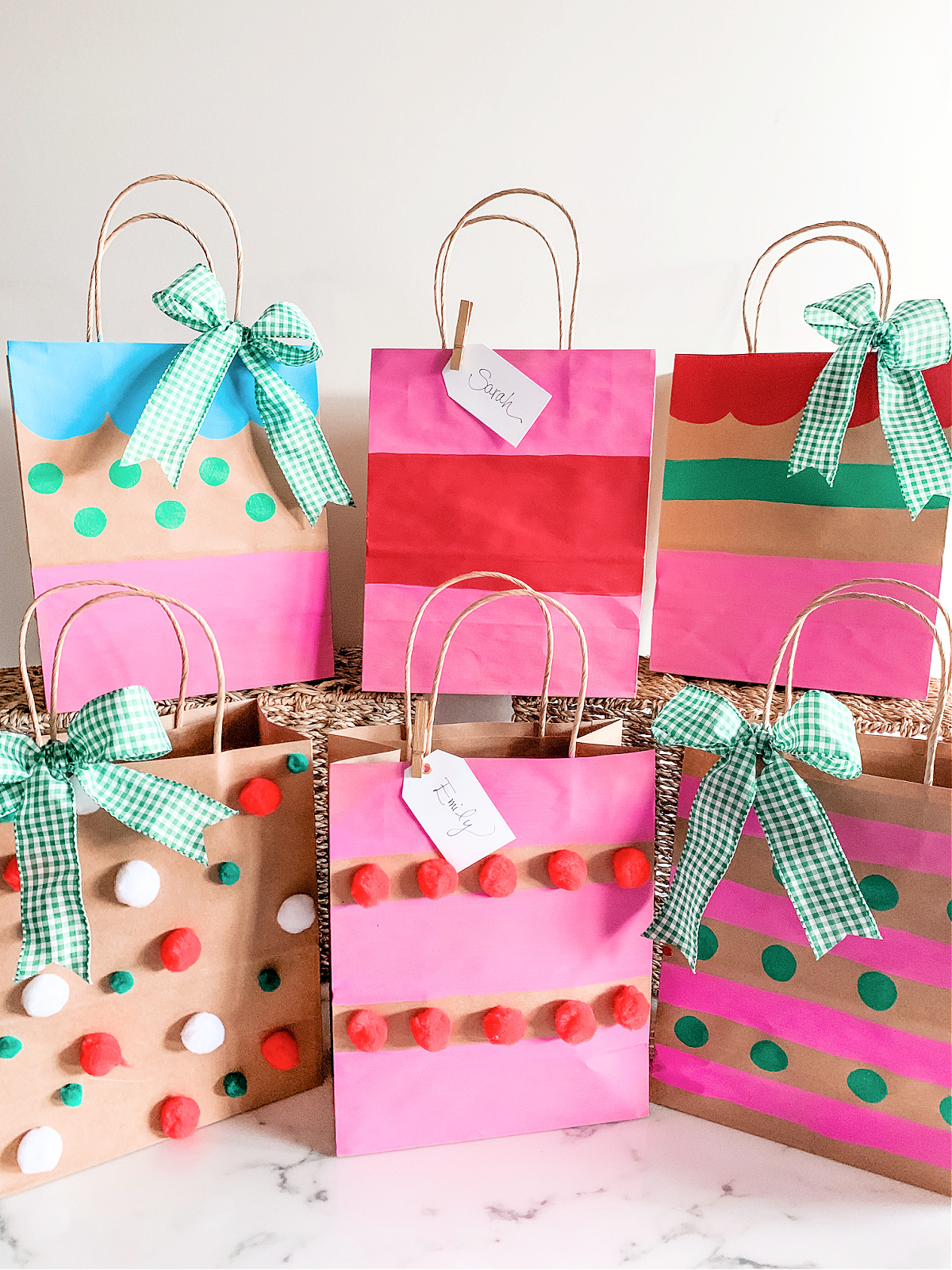The photograph depicts six elegantly decorated gift bags placed against a light stone-colored background, possibly a white marble surface or beige rattan tables. Each bag, made from paper material, features intricate designs with multicolored patterns.

Starting from the top left, the first bag showcases a vibrant look with a light blue top, a beige middle adorned with green dots, and a pink bottom. It is accentuated with a large green checkered bow on one handle. Next, the middle bag at the back has an alternating pink-red-pink pattern, with a white name tag stating "Sarah" clipped on with a paper clip. The third bag in the top row has a striking red scalloped top, a beige middle with a thin green stripe, and a pink base, also featuring a green checkered ribbon on one handle.

In the bottom row, the first bag on the left is decorated with red, green, and white puffballs resembling cotton or gumdrop candies on a beige background, complemented by a green checkered ribbon. The central bag displays a repeating pattern of pink and beige stripes, with two lines of red pom-pom decorations in the middle. This bag has a white label reading "Emily," attached with a clothespin. The final bag on the right has a distinctive design of alternating hot pink stripes and green polka dots on a beige background, finished with a green checkered ribbon on the handle.

All bags are beautifully adorned with ribbons and tags, creating a festive and personalized presentation ideal for gift-giving.